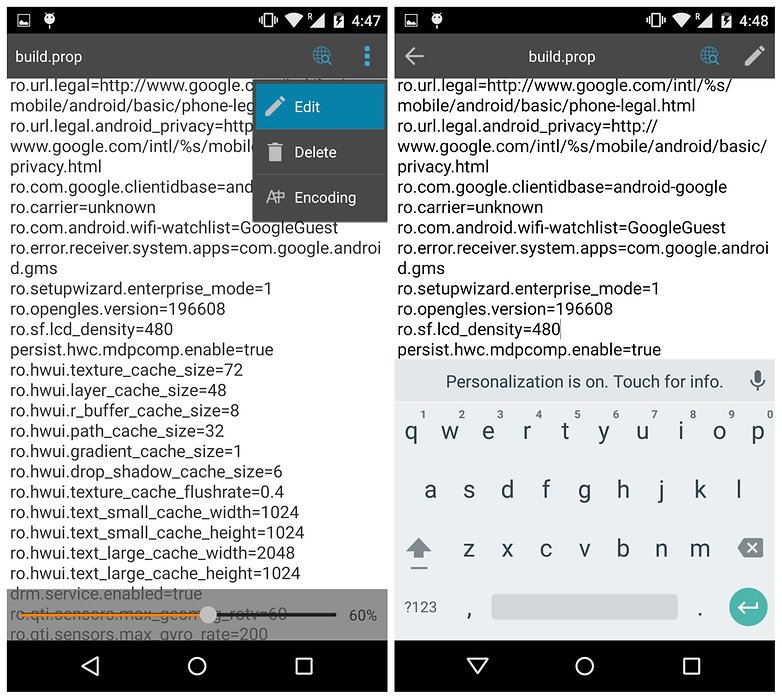The image showcases two screenshots from a mobile device, displayed side-by-side, both containing strings that resemble paths to an online location. Both screenshots feature horizontal blue and black bars framing the top of the images. 

The left image includes an additional pop-up menu with options: "Edit" displayed in white text on a blue background, "Delete" in white text on a gray background, and "Encoding" also on a gray background. 

Meanwhile, the right image has a light gray keypad visible at the bottom, which suggests that text input might be occurring. 

Both screenshots have a white background, indicating that they were taken from the same or similar application interface.